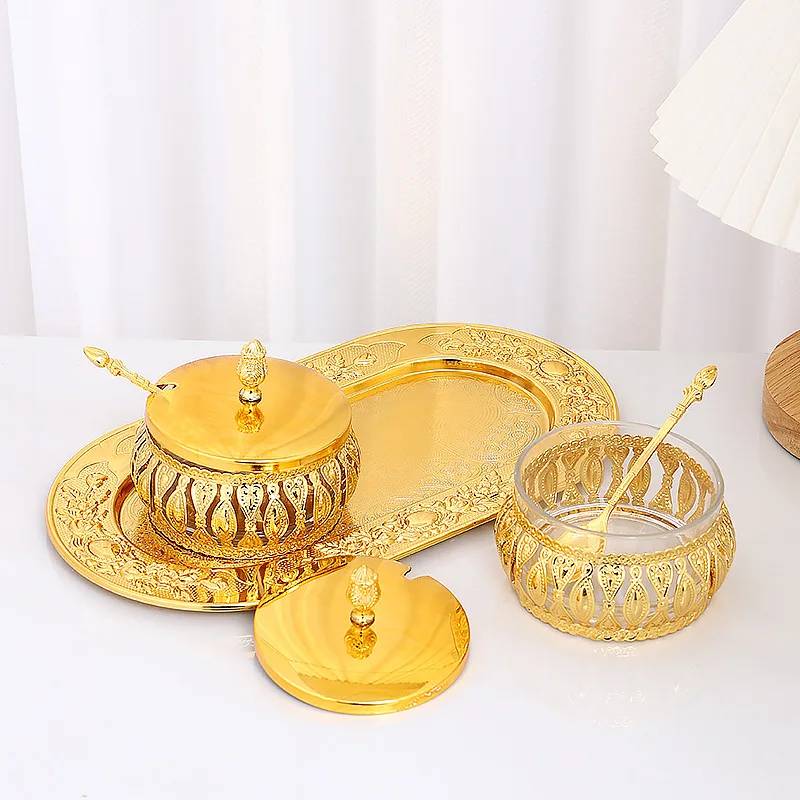The image is a square-shaped indoor photograph, approximately 5 to 6 inches on each side. The lower half features a plain white tablecloth draped over a table or countertop, extending horizontally across the image. Above the table, the backdrop consists of pristine white curtains. In the upper right corner, partially visible is a brown wooden stand of a lamp, with its white, pleated, accordion-style shade extending towards the center and disappearing off the frame.

Dominating the center of the image is an ornate, oval-shaped golden platter adorned with intricate filigree and floral designs. The platter, positioned slightly closer to the lower left corner, holds a round gold bowl. This bowl, exhibiting a shiny gold top with a small hole for a gold spoon, has a translucent red hue indicating it contains some substance. To the right of the tray sits another matching golden bowl, this time off the platter and clearly empty, revealing the glass interior with gold lace-like adornments around the exterior. Its lid lies to the left, showcasing the exposed golden spoon inside.

Overall, the composition features an elegant arrangement of luxurious golden dishware set against a minimalist white background, highlighting the intricate details and reflective quality of the serving set.